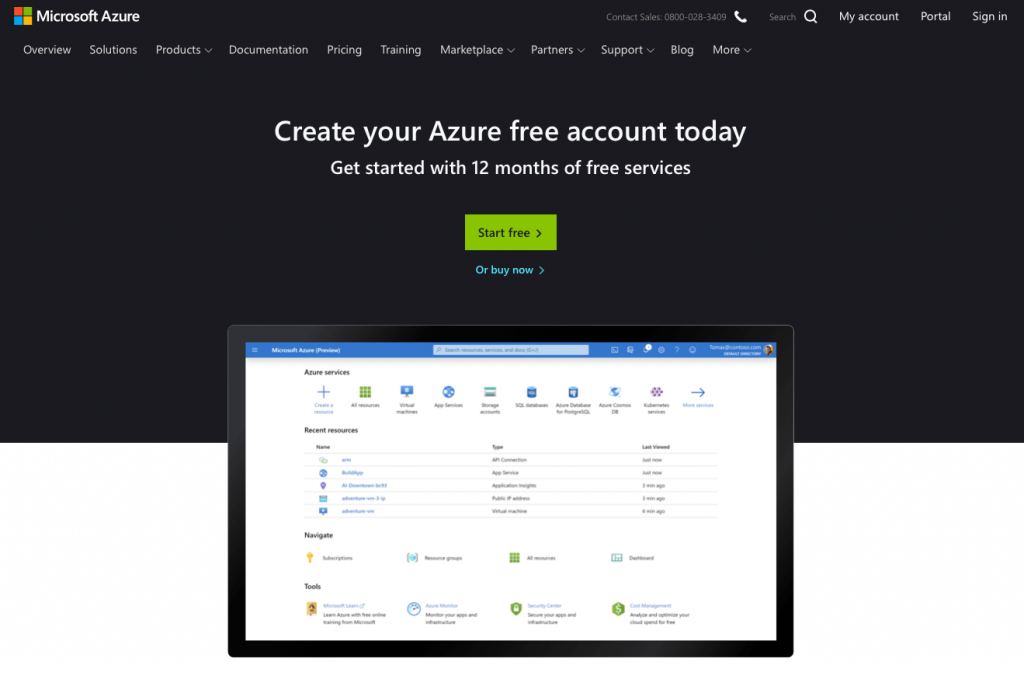A detailed screenshot from a website showcasing Microsoft Azure. The screen is divided into two sections: the top half is predominantly black, while the bottom half is white. Centered within the image is a screenshot of a computer screen. In the top left corner of this screen, the Microsoft Azure logo featuring a multicolored window icon is visible. To the right, there are icons and text links for a phone contact, 'My Account', 'Portal', and 'Sign In'.

Below this header, a navigation menu displays a list of options including Overview, Solutions, Products, Documentation, Prices, Training, Marketplace, Partner, Support, Blog, and More.

The center of the image contains white text that reads, “Create your Azure free account today. Get started with 12 months of free services.” Below this message, there is a green button labeled "Start free" and blue text for "Buy now." Underneath, a depiction of a computer screen shows a blue navigation bar with a search box labeled "Azure services" and a sequence of icons. The screen displays a table with small, somewhat illegible text, followed by a navigation band with various icons and their corresponding text. A tools band, featuring additional icons and text, is visible at the bottom of the screen.

The detailed layout and promotional messaging suggest the image is part of an introductory or signup page for new Microsoft Azure users.